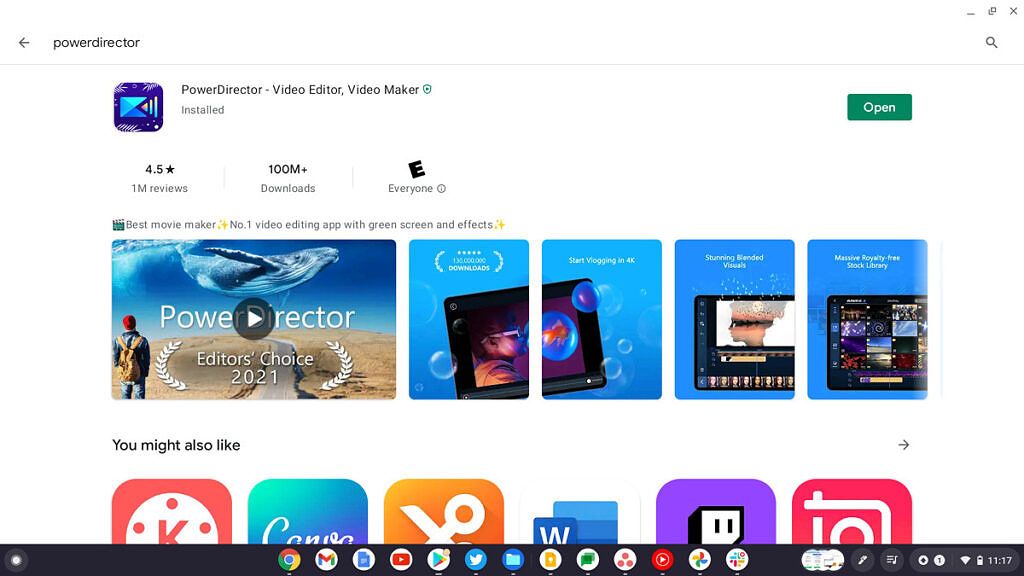The image captures a close-up view of a smartphone or tablet screen as someone browses a selection of apps. The user appears to be considering opening the PowerDirector app, prominently displayed in the top left corner. The full name of the app, "PowerDirector Video Editor, Video Maker," is clearly visible along with a small green 'Open' button on the right-hand side, indicating that the app is already installed on the device.

A search icon is located opposite the PowerDirector name at the very top of the screen, suggesting the user can search for other apps if needed. Below the PowerDirector icon, additional details reveal that the app has garnered 1 million reviews, boasts a 4.5-star rating, and has been downloaded 100 million times, reflecting its popularity and user satisfaction.

Further down the screen, a series of four thumbnail screenshots showcase the app's features and interface, complemented by a demonstration video on the left-hand side. Beneath these visuals, there are suggestions for similar apps, each represented by their respective icons. At the bottom of the screen, a row of icons indicates other applications that the user frequently accesses, providing a glimpse into their app usage habits.